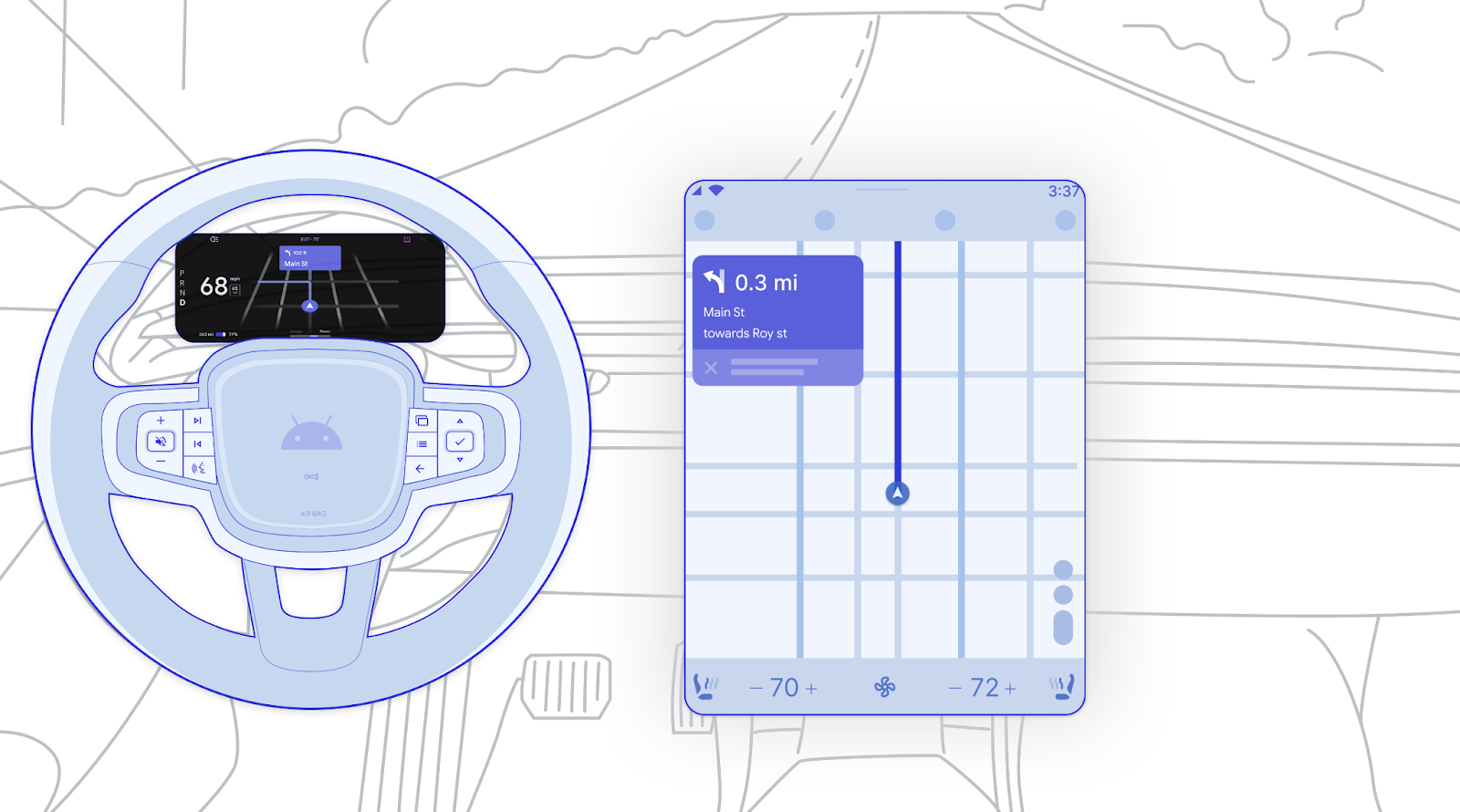The illustration showcases the interior view from the driver's seat of an automobile. The focal point is the integrated technology within the car. The steering wheel, positioned on the left, features an Android logo and is detailed with various controls, including volume, track navigation, and other multimedia buttons. Above the steering wheel, embedded in the inner circle area, is a black screen displaying speed, street information, and navigation data. The center console hosts a large tablet-like display that provides a map with turn-by-turn directions, indicating an upcoming left turn in 0.3 miles onto Main Street. The simplistic, gray-lined depiction of the dashboard contrasts with the distinct blue lines of the steering wheel and elements of the center console. Through the windshield, the scene reveals an open two-lane road flanked by faint outlines of trees, with no other vehicles in sight, emphasizing the route straight ahead. The composition and technology suggest a modern, perhaps Android-integrated vehicle designed for a smooth and connected driving experience.